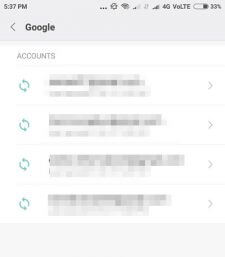The image appears to be a low-quality screenshot or screen recording from a mobile device. At the top, the time is displayed, likely showing "5:37 PM," followed by three dots and various icons indicating phone status such as a signal icon, "4G voLTE," and a battery icon displaying approximately 33% charge. A gray box at the top contains a back arrow, the bold text "Google," and the gray text "Accounts." Below this header, there are four entries with pixelated text, each accompanied by a blue-green refresh icon on the left and a gray arrow on the right, suggesting these entries are clickable. These blurred entries likely represent account names linked to Google on the device. The layout and interface strongly indicate that this screenshot is from the settings menu of an Android phone, specifically within the Google account management section.